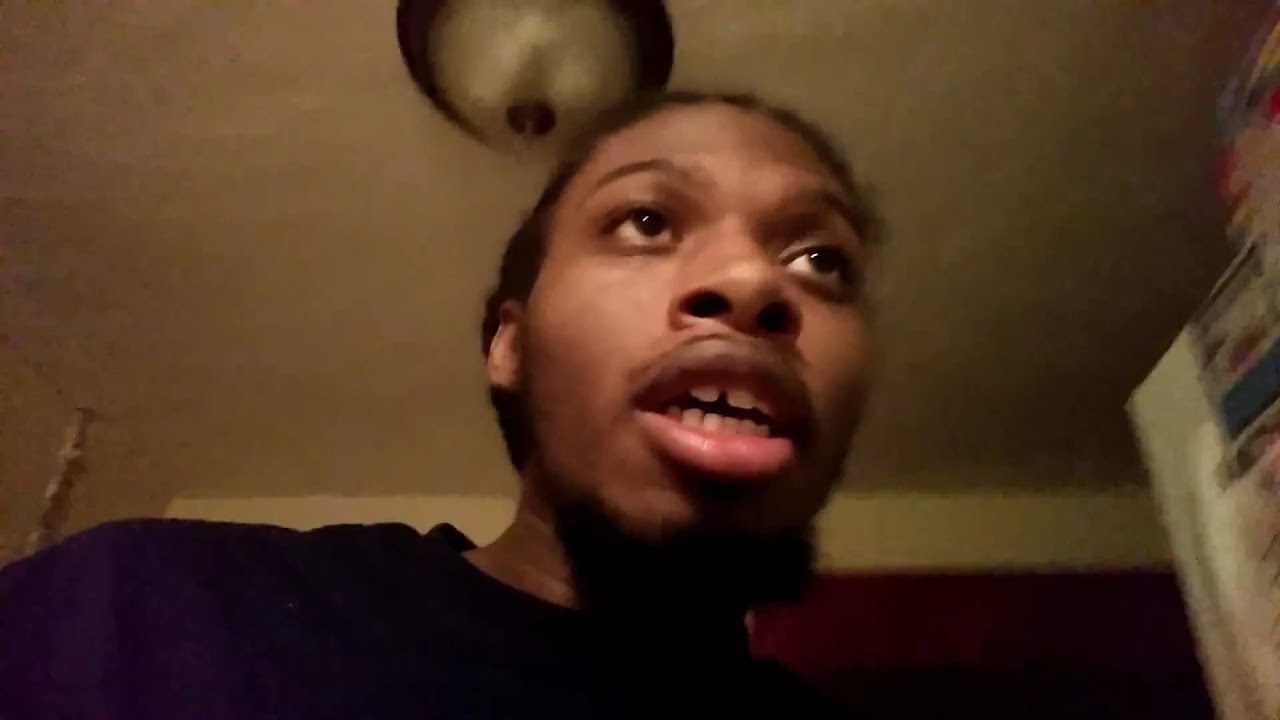This photograph features a young, dark-skinned man in an indoor setting, likely within a room of his house. The man’s face and shoulders dominate the frame, with his eyes gazing upwards and his mouth slightly open, revealing both rows of white teeth as if he is about to speak. He has short black hair, dark eyes, and a neatly trimmed beard primarily on his chin, along with dark brown eyebrows. He wears a dark navy blue shirt. The background, slightly blurred, shows a white ceiling adorned with a domed-shaped light fixture that has a black or brown base. Part of a red wall is visible, along with some indistinguishable images containing colors such as white, blue, red, and black. There's also a post, possibly from a bed, and what seems to be a closet or a door on the right side of the image.